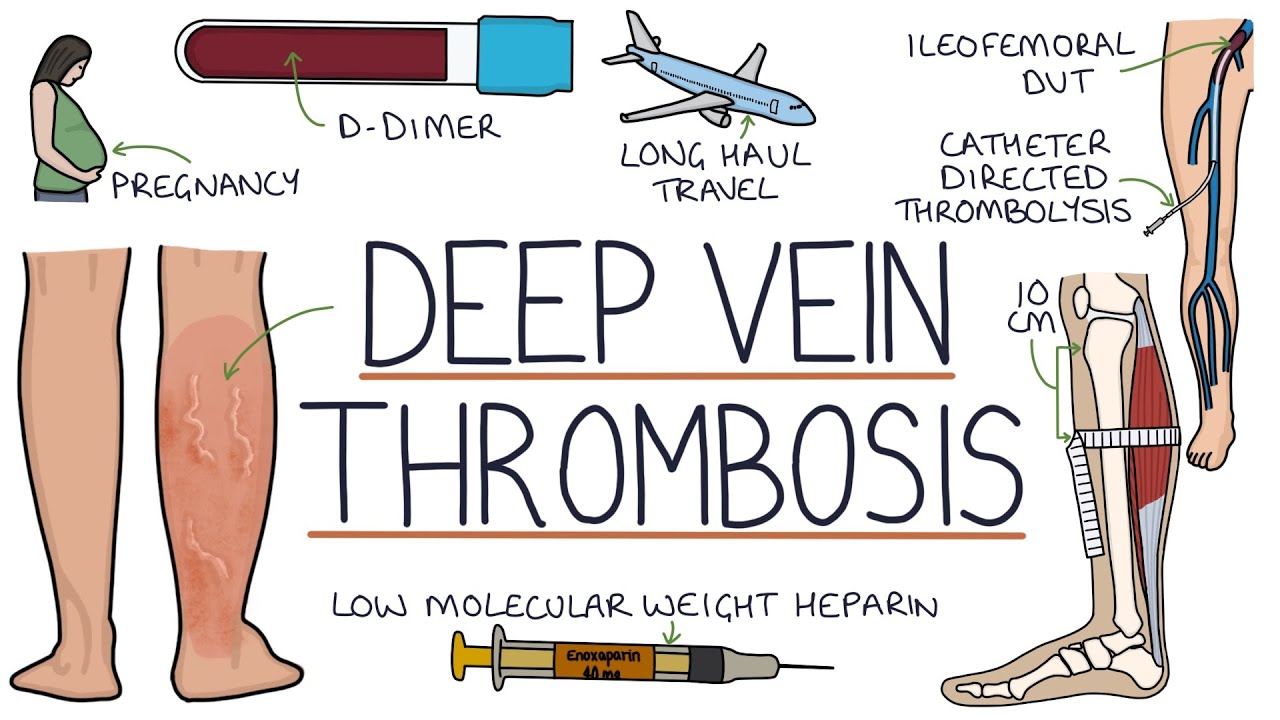This colorful, cartoonish medical infographic illustrates various aspects and causes of deep vein thrombosis (DVT). Prominently, it features a pregnant woman holding her belly in the upper left, signifying pregnancy as a risk factor for DVT. Below this, there's a maroon-red test tube labeled "D-dimer," indicating a blood test used in diagnosing DVT. Adjacent to these is an image of a jet airliner, drawing a connection to the risk of DVT associated with long-haul travel.

In the center and lower sections, detailed drawings of human legs show the internal veins and the effects of DVT. One noteworthy illustration presents veins and a catheter performing directed thrombolysis—highlighting a medical intervention. Another detailed image on the lower right shows a cross-section of a calf, with off-white bones, red muscles, and fleshy skin, including a 10-centimeter measurement likely for diagnostic purposes. The veins coming to the surface of the calf and muscle structure are also emphasized.

Finally, a syringe at the bottom labeled "low molecular weight heparin" suggests the medication used for treating DVT. The infographic altogether provides a comprehensive visual representation of the causes, diagnosis, and treatments associated with deep vein thrombosis.